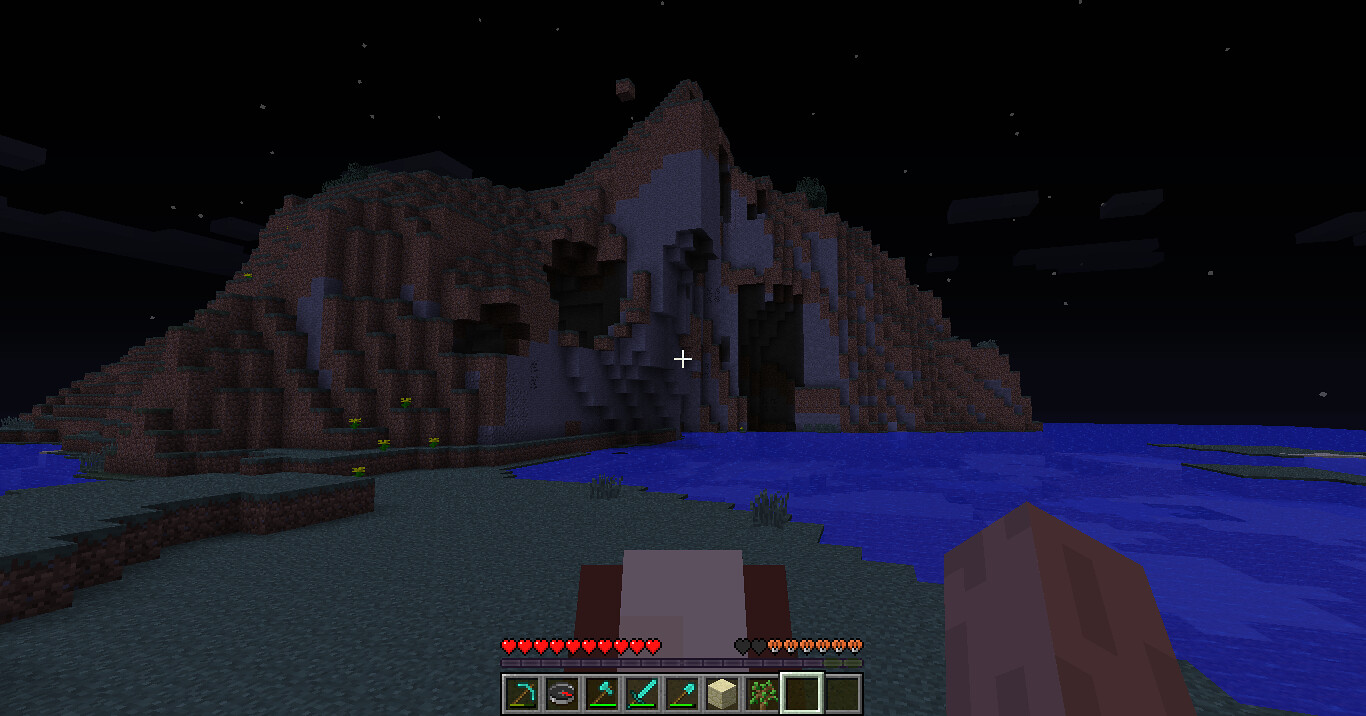This nighttime Minecraft screenshot, captured from a landscape orientation, portrays a serene yet intriguing scene. The dark, star-studded sky serves as a backdrop in the top half of the image. In the foreground to the right, a body of water displays two shades of blue—a darker base with lighter patches. The shore, situated to the left and extending to the center, features blocks of green grass organized on two distinct levels with some plants scattered across it.

Dominating the distance is a gray and brown mountain, home to three caves: a tall one descending towards the water and two smaller ones higher up. The base of the mountain is adorned with yellow flowers, adding a splash of color to the otherwise muted landscape. Small islands dot the water, contributing to the scene's complexity.

In the immediate foreground, the player's inventory is visible at the bottom center of the screen, showing an array of weapons and tools. Above the inventory slots, a row of roughly 10 red hearts indicates the player's health, while additional small orange and pale green icons hover next to them.

The image also captures the player's arm or tool in action on the right side, emphasizing the immersive and interactive nature of the game.